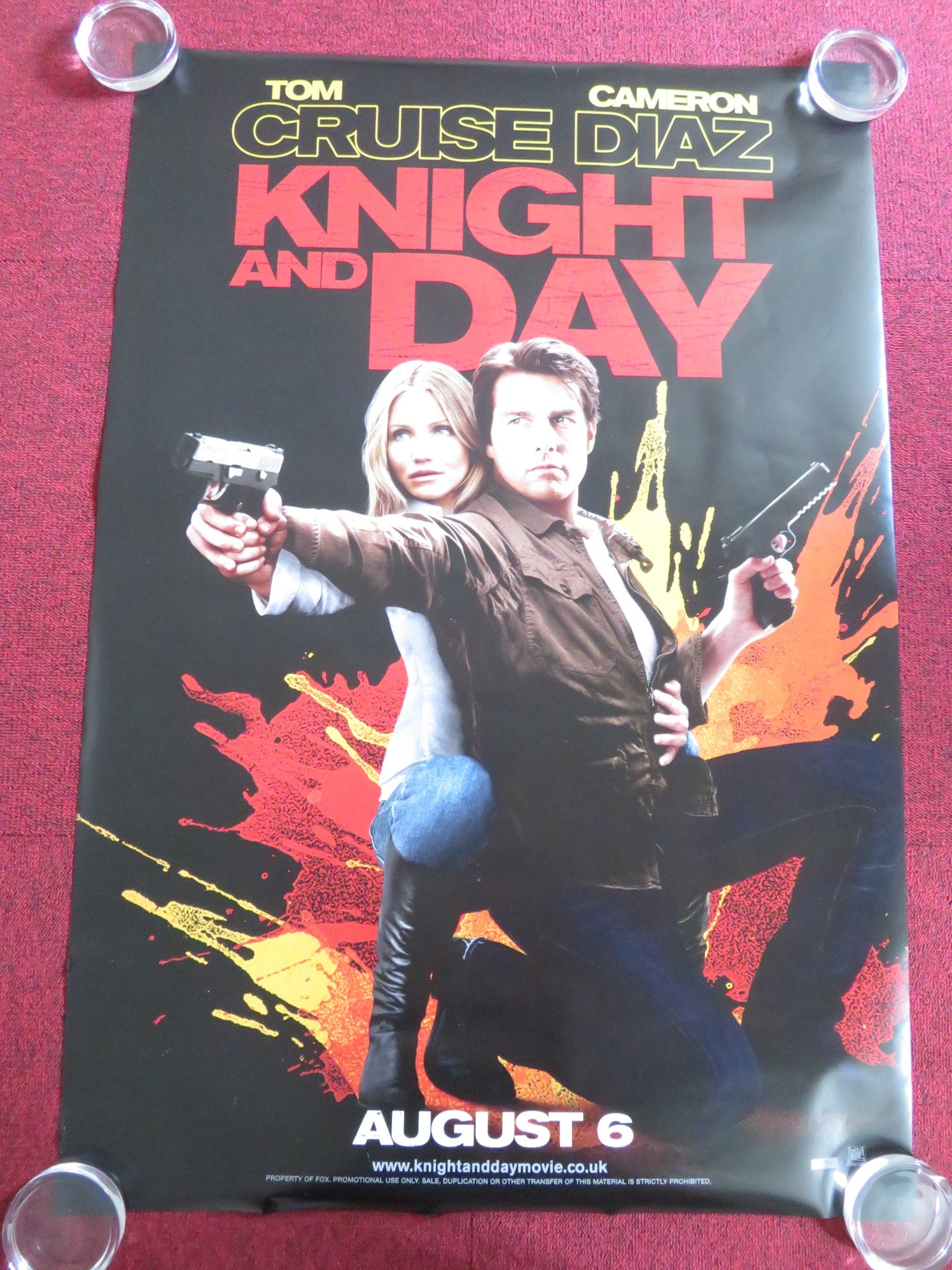The image depicts a movie poster for "Knight and Day" featuring Tom Cruise and Cameron Diaz. The poster is laid out on a purple or maroon pink carpet, being held down at its four corners by clear round glasses or weights to prevent it from rolling up. The background of the poster itself is predominantly black. Tom Cruise and Cameron Diaz are prominently displayed in the center; Cruise is holding a gun in his right hand with a straight arm, while Diaz is positioned closely behind him, also gripping the gun. Behind them, a vibrant explosion-like splotch of red, yellow, and orange paint adds dynamic energy to the scene. The actors' names, "Tom Cruise" and "Cameron Diaz," are printed at the top of the poster. The movie's title, "Knight and Day," is highlighted in bold, bright red letters, standing out strikingly against the dark background. At the bottom of the poster, the release date, August 6th, is presented in white letters. Additional, smaller text provides more details about the movie, although it is hard to read. The color palette of the poster includes black, red, orange, yellow, white, blue, and silver.